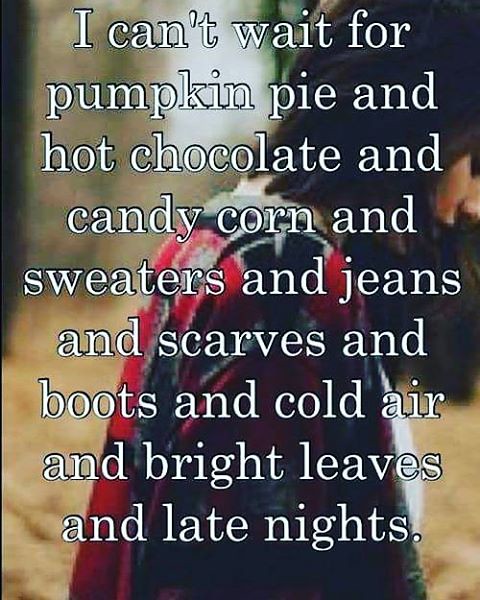The image depicts a woman with black hair that extends just past the nape of her neck, walking along a path carpeted with yellow leaves. She is wearing a sweater with black, gray, and red tones and appears to be deep in thought, looking down at the ground. Positioned slightly to the right in the frame, the woman gives a sense of introspection amid an autumnal backdrop. The background features blurry trees, emphasizing the fall setting. Overlaid on the image, in white serif font with a shadow effect, is the text: "I can't wait for pumpkin pie and hot chocolate and candy corn and sweaters and jeans and scarves and boots and cold air and bright leaves and late nights." The image quality is somewhat degraded, giving it a nostalgic, almost poetic feel, often associated with social media meme-style graphics celebrating the essence of fall.